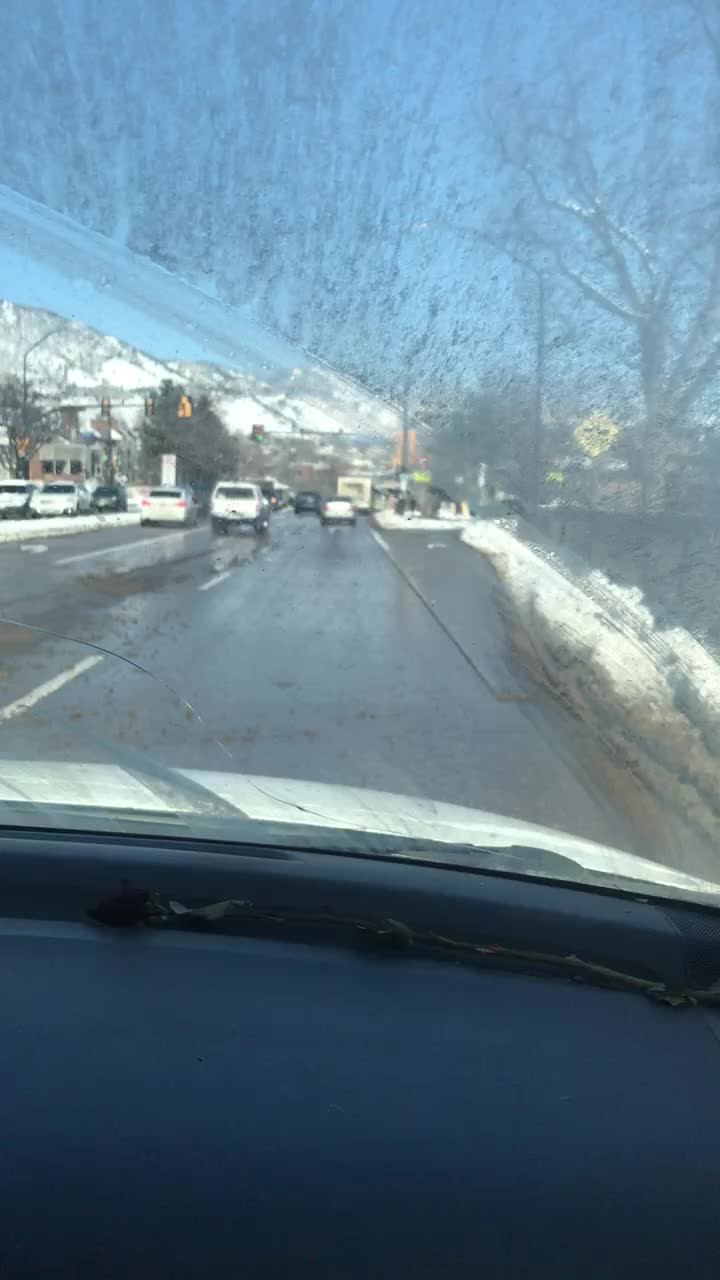A vertically-oriented photograph taken from the passenger side of a car, looking out through a dirty front windshield. The windshield wipers have cleared a patch, contrasting starkly with the grimy sections outside their reach. The street ahead is wet and slightly blurry, bordered by modest piles of snow on either side. Several cars line the street, leading toward the background where a streetlight stands vigil. In the distance, snow-capped modest mountains rise beneath a perfectly clear blue sky, flanked by buildings and trees that hint at a crisp, cold day. The front of the car, painted white, is faintly visible at the bottom of the image.